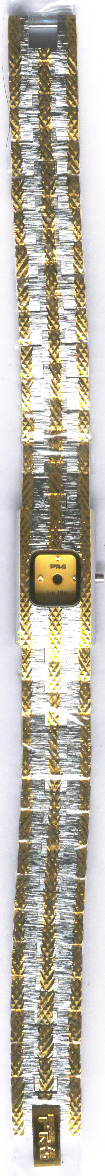This image features a tall, slender electronic component set against a white background. The component closely resembles a watch strap in its form. The main band of the piece is a whitish-silver color, edged elegantly with gold on both sides. Additionally, a gold stripe runs down the middle of the band, adding to its intricate design. In the center of this band, there's a prominent orange square that houses a black circle, framed by a thin black border, adding a striking contrast to the otherwise metallic tones. At the top of the component, a small clasp is visible, resembling those found on traditional watch straps. At the bottom, there appears to be a gold insignia with some letters, although the exact details are difficult to discern.